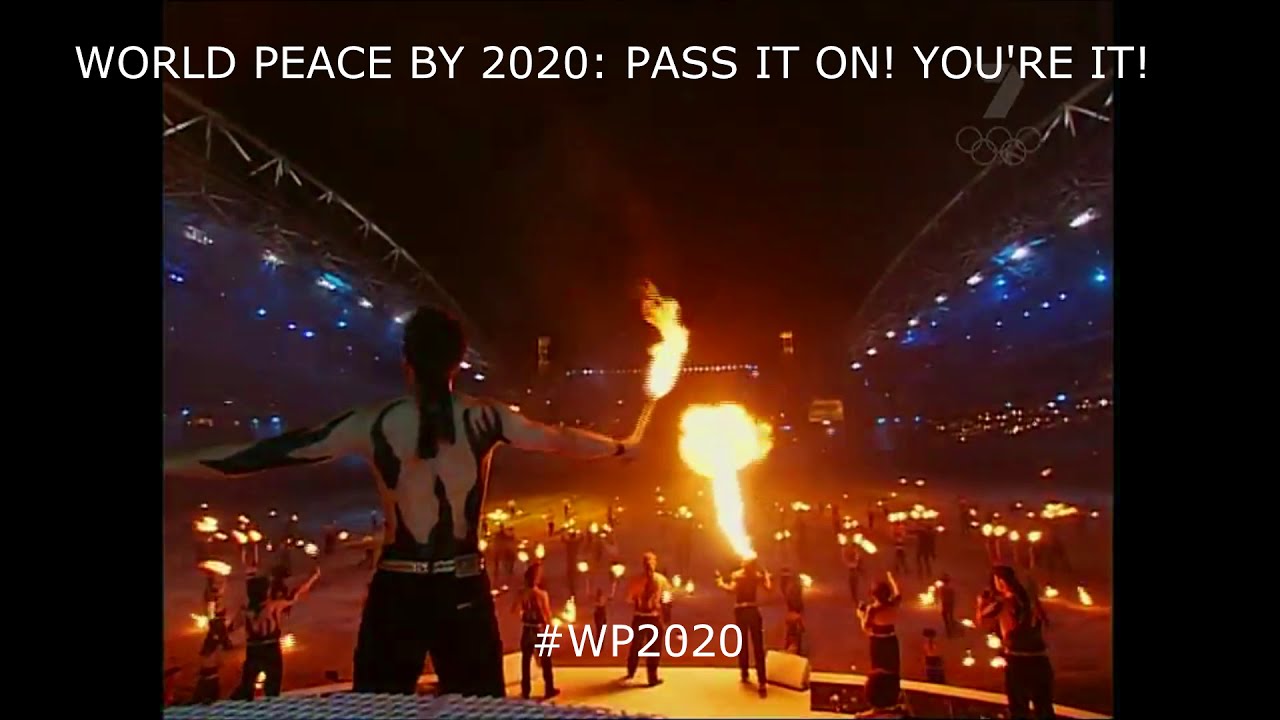The image appears to capture a dynamic and captivating performance at an outdoor stadium event. Taken from the back of a stage, it showcases multiple performers holding flaming sticks, engaging in fire dancing acts. The stage is bustling with activity, dominated by individuals clad in black body paint and black pants, contributing to the dramatic visual effect. In front of the stage, a performer is impressively blowing fire from their mouth, adding to the thrilling atmosphere. The background features dark, almost black surroundings with blue lighting, and the setting appears to be a vast arena with an open roof, packed with spectators on both sides. Overhead, the message "World Peace by 2020, pass it on, you're it" is prominently displayed in white font, with the hashtag "WP 2020" centered at the bottom of the image. Adding to the mesmerizing visual palette, the scene is filled with hues of black, blue, orange, yellow, and various earthy tones. In the foreground, performers continue their fire tricks on the ground, illuminated by the flickering flames and casting an impressive display against the nighttime sky.